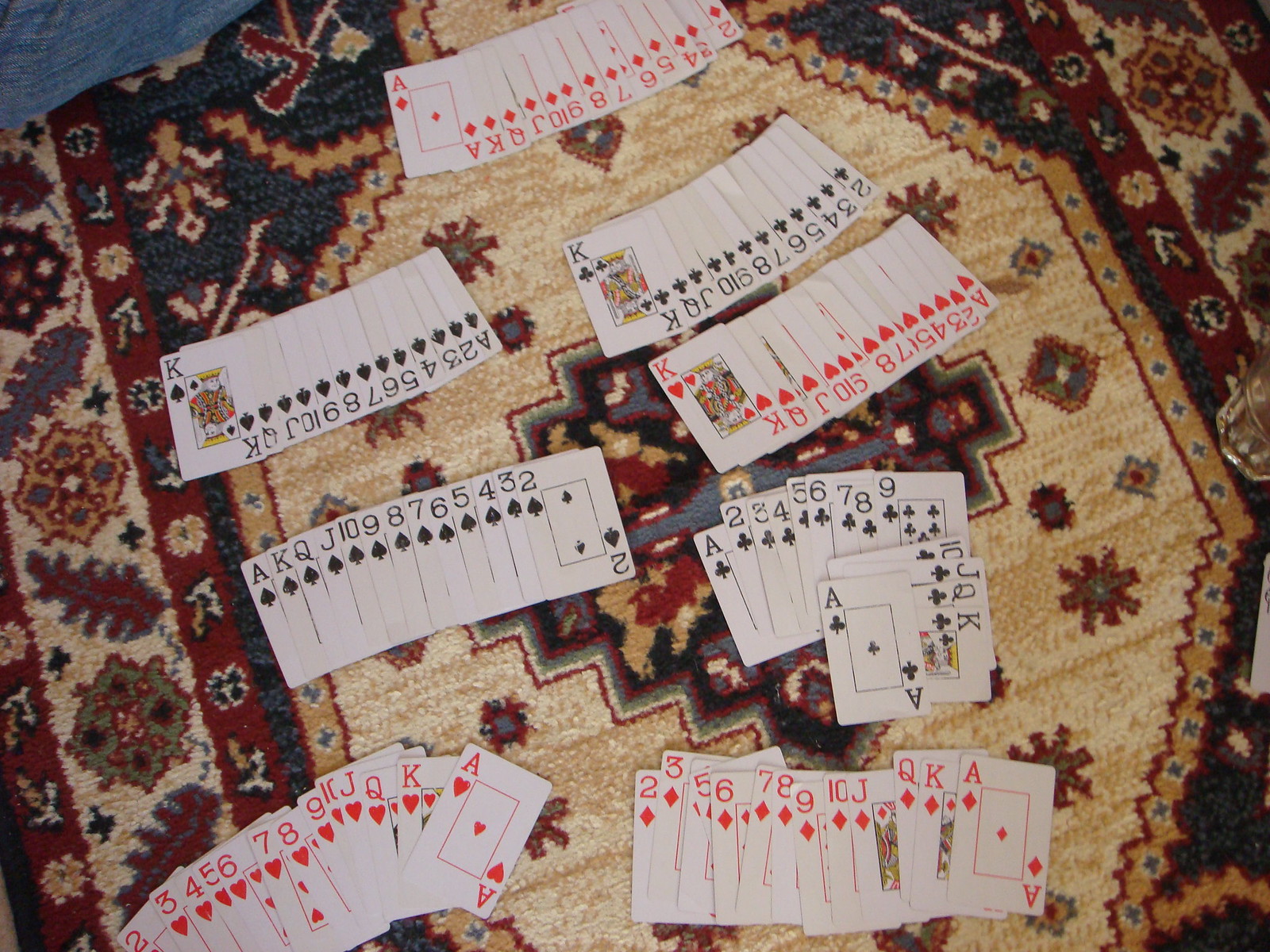This vibrant color photograph offers a top-down view of a dazzling Persian rug, adorned with intricate designs in shades of gold, maroon, and dark blue. The rug features a large, central gold octagon that captures immediate attention. Neatly placed atop this elegant rug are playing cards, meticulously arranged by suit.

At the top center of the composition, the suit of Diamonds is showcased in perfect sequence from left to right: Ace, King, Queen, Jack, 10, and so forth. Directly below, the suit of Clubs is arranged on the right side, starting from the King and moving leftward through Queen, Jack, 10, 9, and beyond. Adjacent to the Clubs on the right side, the Spades begin with the Ace and continue in a similar orderly fashion.

As we move our gaze downward, another line of Clubs is visible, this time aligned in a left-to-right order from Ace to King, Queen, Jack, 10, and so on. The bottom left-hand corner introduces the suit of Hearts, organized right to left: Ace, King, Queen, Jack, continuing sequentially. The right side opposite this features the suit of Diamonds, also in right-to-left order with the same progression.

Above this section, the Clubs make another appearance, in a similar format. Just above the Clubs, another display of Hearts is shown, arranged from right to left in increasing order starting from the Ace, followed by the 2, 3, 4, 5, and continuing upwards. Finally, the upper right-hand corner shows yet another set of Clubs, ordered from King, Queen, Jack, and onwards, though noticeably missing or hiding the Ace.

The entire composition not only highlights the exquisite craftsmanship of the Persian rug but also the meticulous organization of the playing cards, offering a visually rich and stimulating tableau.